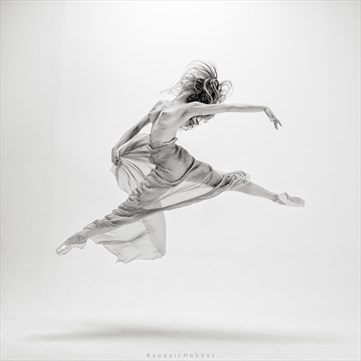This square image features a detailed and elegant black and white rendering of a mid-air ballerina against a bright, silvery-white background. The ballerina is captured in a dynamic split leap, with her left foot pointing towards the lower left corner and her right foot pointing above the lower right corner. Her long, messy hair flows freely as her head tilts back, partially obscuring her face. She is topless and has a long, transparent dress draping over her lower body. Her left arm stretches backward, while her right arm extends forward, grasping the edge of the flowing fabric. She wears ballerina slippers, and a shadow is visible beneath her, emphasizing her airborne movement. Overall, the drawing highlights the grace and fluidity of her dance in a striking, monochromatic palette.